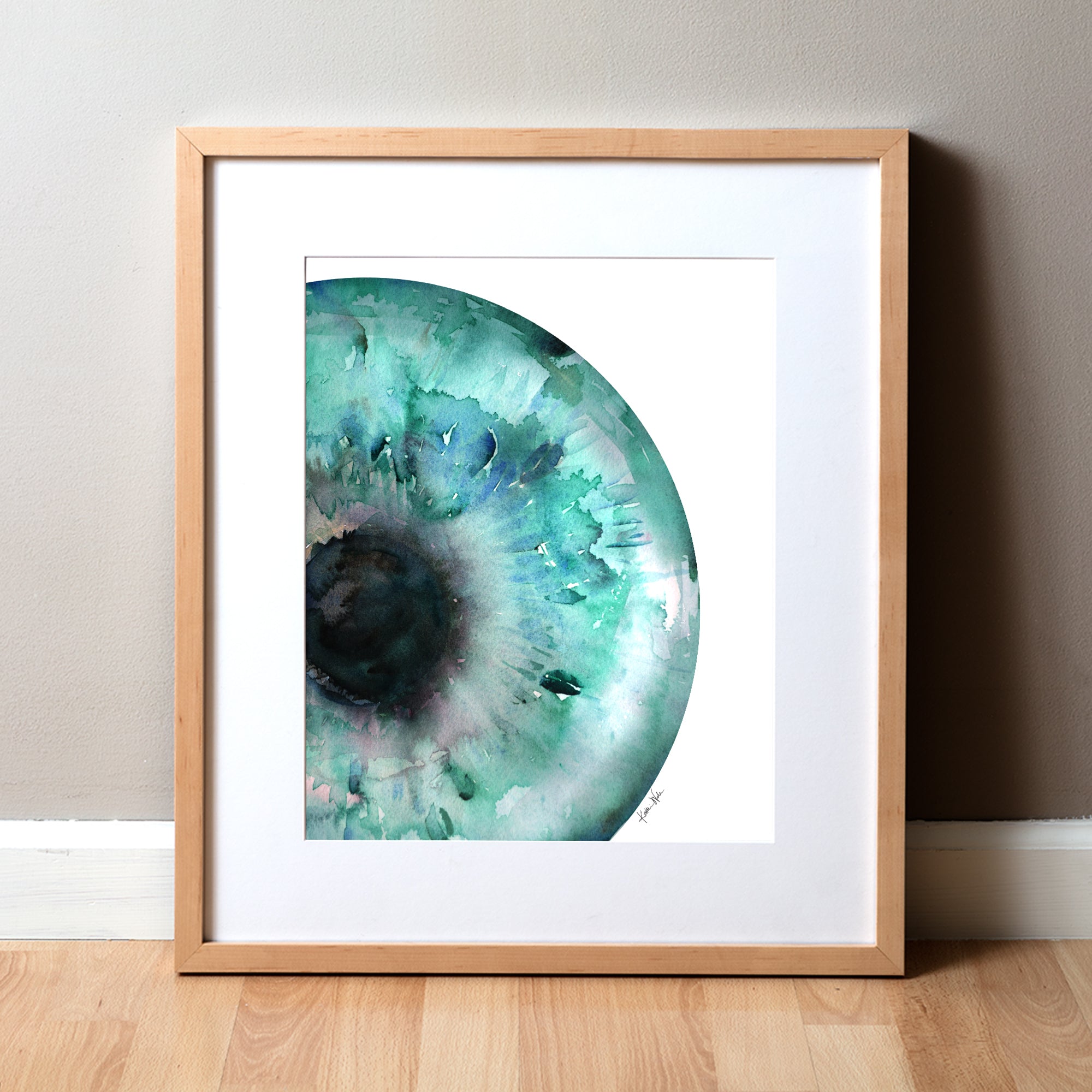The image depicts a photograph of a framed painting leaning against a gray wall with white trim, set on a hardwood or possibly light wood vinyl floor. The painting itself is encased in a light brown wooden frame with a white mat. The artwork appears to be an extremely close-up and somewhat ambiguous depiction of a human eye, although it could also be interpreted as something else due to the abstract nature of the piece. The central feature is a large, dark circle resembling a pupil, located slightly below the center and to the left. Surrounding it is an iris-like area rendered in a splotchy watercolor style, incorporating vibrant shades of blue, green, and white, with hints of deep purple. There are no distinct striations typically found in an eye, enhancing its abstract quality. The background of the painting is completely white, providing a stark contrast to the colorful central image. In the lower right corner of the possible iris area, there is a small artist's signature, which is too small to be legible. This piece, potentially for sale online, presents a striking metaphor, possibly representing an eye or the Earth, or even both.